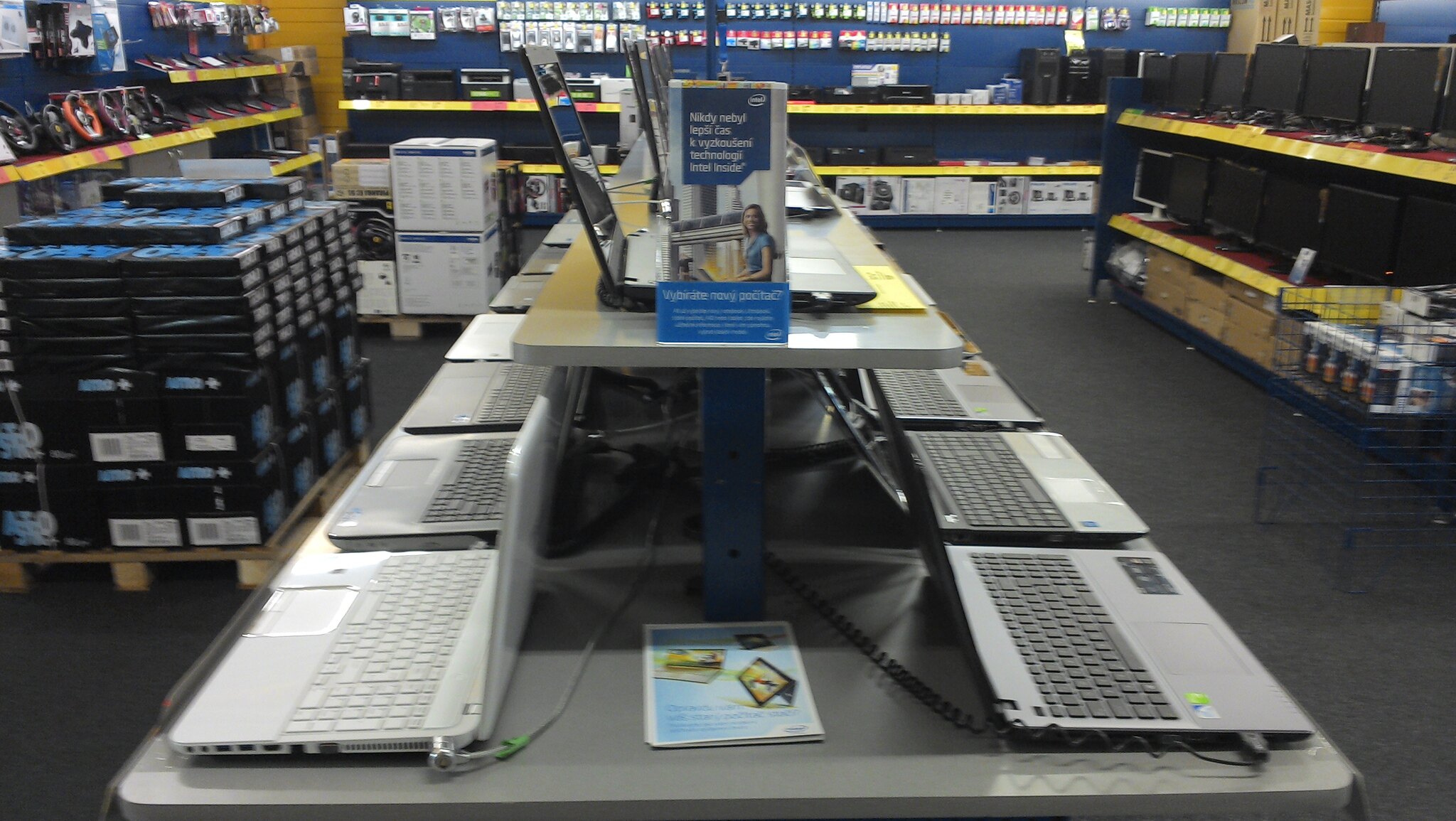This photograph depicts the interior of a Best Buy store, featuring a detailed display of various electronic devices. Dominating the scene is a long, central countertop that runs from the front to the back of the image, lined with rows of laptops on either side, each secured by security cables. Above these, a raised middle shelf also holds a row of laptops and an assortment of pamphlets, one of which lies at the front of the display and another placed on this upper level. The background features a characteristic blue wall adorned with hanging merchandise, while the shelves exhibit bright yellow edges that draw attention. To the left, there is a noticeable palette of printer paper alongside a display of headphones. To the right, multiple shelves showcase computer monitors and their boxes, with additional printers and ink cartridges visible towards the back of the store. The photograph has a dimmed, desaturated look, with overhead lighting providing subdued illumination, giving the entire scene a slight gray cast.